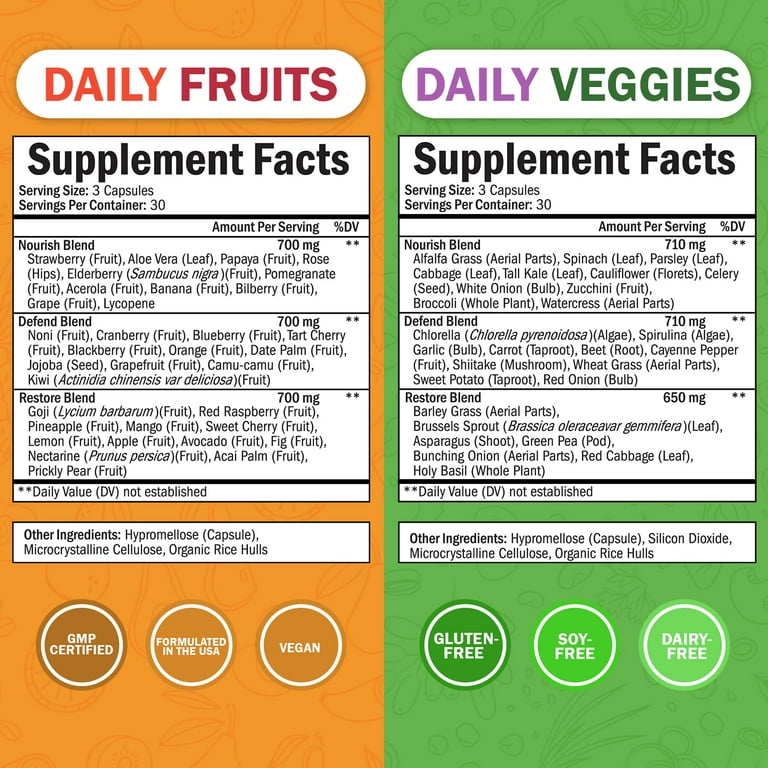The image depicts a detailed nutrition label divided into two distinct sections with vibrant colors. The left side has an orange background and is labeled "Daily Fruits" in an orange and maroon font. The right side features a bright green background labeled "Daily Veggies" in a purple and dark green font. Both sections are topped with a white, pill-shaped header that spans across the top of both colors.

Below each header, the text "Supplement Facts” appears, detailing that the serving size is three capsules, with 30 servings per container. There are three blends listed under each section: the Nourish Blend, the Defend Blend, and the Restore Blend, each composed of various ingredients. For the fruit section, notable ingredients include strawberries, papaya, rose hips, elderberry, pomegranate, aloe vera (leaf), and bilberry. 

The colors used in the design include shades of orange, purple, dark red, darker orange, green, light green, lime green, dark green, white, grays, and blacks, creating a vibrant yet organized visual structure.

At the bottom of the label, certification icons are displayed. On the left side (Daily Fruits), features include "GMP Certified," "Formulated in the USA," and "Vegan" in white text inside white circles. On the right side (Daily Veggies), icons denoting "Gluten Free," "Soy Free," and "Dairy Free" are rendered in green circles with white borders.

Overall, this label provides a comprehensive overview of the dietary supplements, emphasizing ingredient transparency and certification credibility.